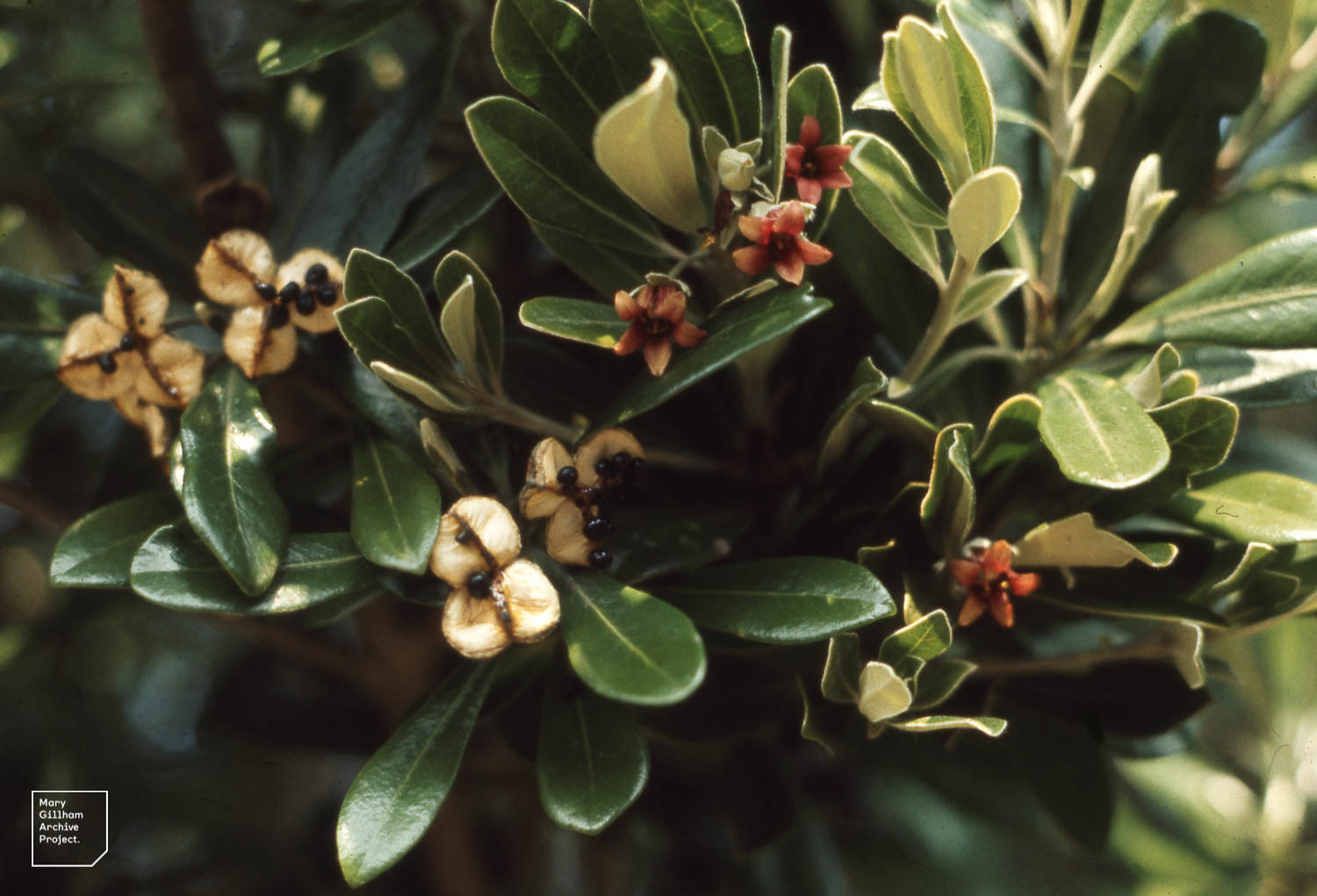This is a close-up photograph of a small plant with lush, thick green leaves that are shiny and appear almost white on the right side due to a light source. The background is blurred and dark, highlighting the plant in the foreground. This plant features multiple thick green leaves as well as other botanical elements, including various flowering parts. On the left side, there are rounded yellowish leaves adorned with small black dots, reminiscent of banana slices with seeds. Also, scattered throughout the plant are small, star-like flowers with five pink petals and black centers. Toward the middle, there are clusters of flower buds and beige, paper-like seed pods with black seeds. The bottom left corner of the image displays a distinct watermark: a five-sided square with one corner clipped off, containing the text "Barry Glibson Archive Project" in white font.